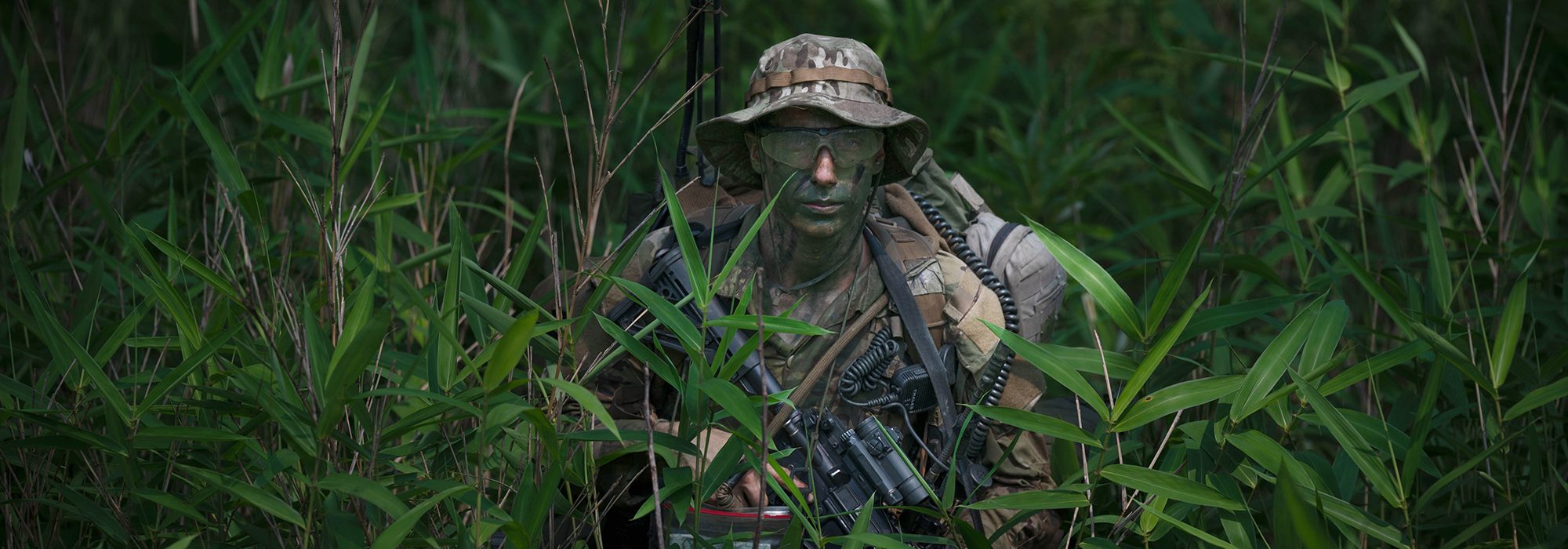In this detailed widescreen photograph, a soldier is crouching amidst tall grass and weeds, blending seamlessly with his surroundings. He is dressed in a full camouflage outfit, including a bucket hat with a brown band and translucent safety goggles that obscure his eyes. His face is painted in dark green and black camouflage, with only his nose and lips standing out in pink hues. The soldier, who appears to be in a wooded area, has his upper body obscured by dense vegetation that dominates the image's left and right thirds. 

Equipped with various gear, his uniform features a radio with a coiled cable attached to a brown strap over his left side. The rear half of a gun is visible, with its black stock forming a triangle over his right shoulder and a barrel scope peeking out to the right. The dominant colors in the image are shades of green and brown, enhancing his camouflage amidst the greenery. The posture and context suggest he is on a mission, possibly lying in wait, perfectly blending into the natural surroundings.